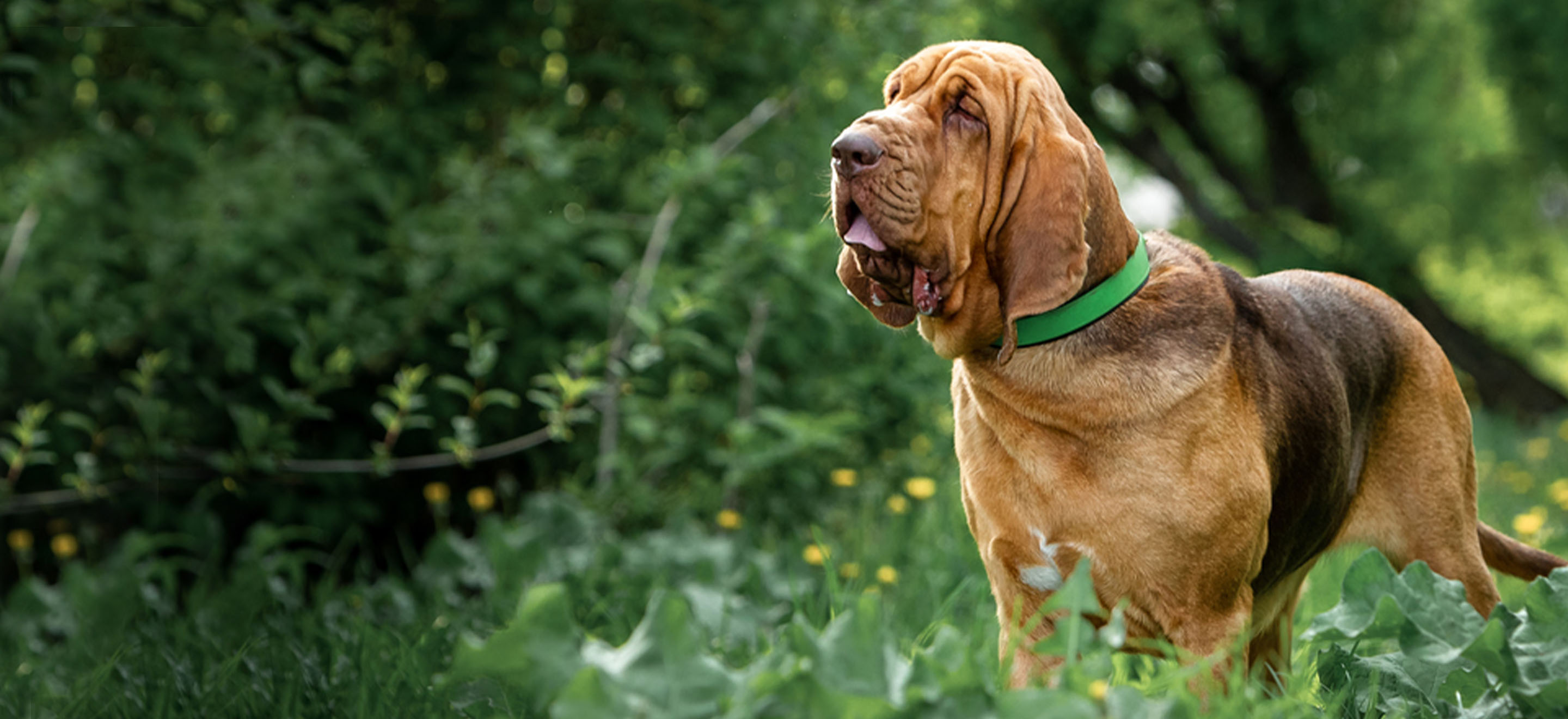In this detailed image, we see an old basset hound with distinct physical characteristics, standing in a lush, green, grassy field. The hound, sporting a green collar, has a rich coat of brown and tan with black patches across its back and belly. Its face is adorned with loose, sagging skin and long, hanging ears that emphasize its aged appearance. Droopy jowls and visible drool contribute to the overall impression of its tired, worn-out expression. The eyes, partly open and partly closed due to the drooping skin, add to its melancholic demeanor.

The field is vibrant with greenery, filled with various plants and trees, their green leaves forming a dense backdrop. Brown and gray branches interlace through the vegetation. Scattered throughout the scene are bright yellow and purple flowers, offering bursts of color amidst the verdant setting. This charming hound, positioned at the edge of the frame, stands amidst this picturesque natural scenery, either resting or possibly gearing up for a hunting escapade in its serene habitat.